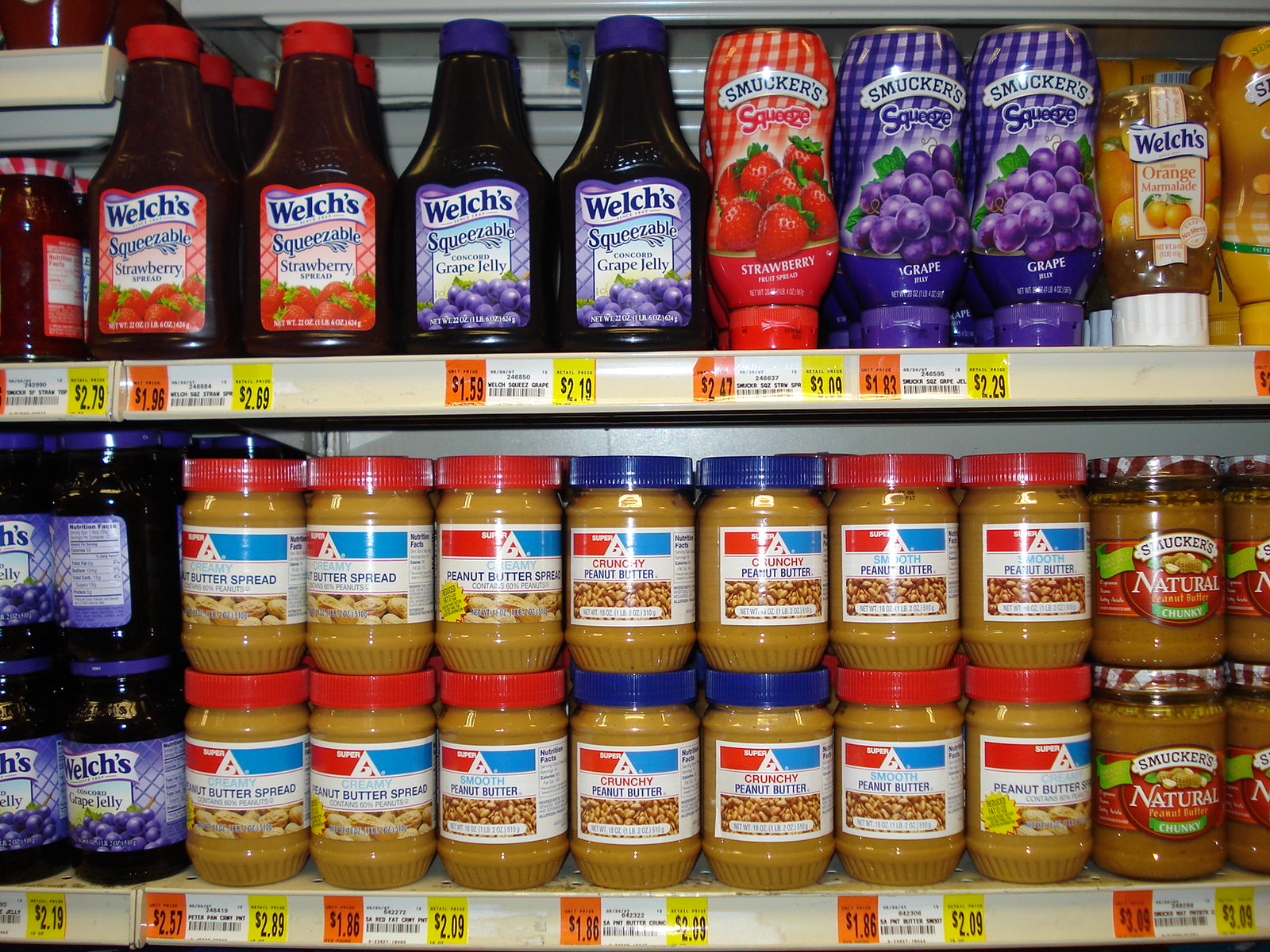A large square photograph captures a section of store shelves stocked with various jellies and peanut butter. The top shelf prominently features an assortment of jellies. On the left side of this shelf, a collection of glass jars filled with various types of jellies is neatly arranged. Dominating the center of the top shelf are a range of plastic bottles containing jelly from well-known brands like Welch's and Smucker's. Below, on the second shelf, starting from the far left, there are several jars of Welch's grape jelly. The rest of this second shelf, spanning the entire center to the right, is filled with an assortment of peanut butters in different varieties and brands. The price tags for these products are visible on the lip of the metal shelves, both on the top and bottom rows. Additionally, in the top left corner of the image, the edge of an adjacent shelf is partially visible, suggesting the continuation of the store's wide selection of products.